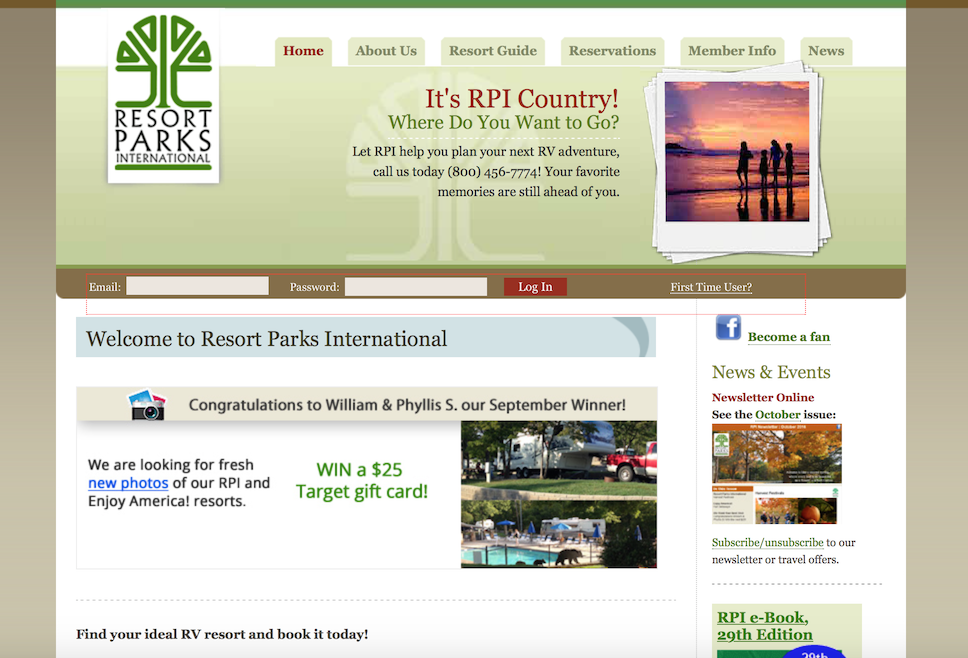The image features a colorful landscape-oriented website promoting Resort Parks International. The site has a simple but clean design, although not overly sophisticated. At the top of the page is the Resort Parks International brand logo, depicting a green, minimalist cross-section of a tree.

The website header includes navigation tabs for Home, About Us, Resort Guide, Reservations, Member Info, and News. The main area of the homepage has large text that reads, "It's RPI Country. Where do you want to go? Let RPI help you plan your next RV adventure. Call us today at 800-456-7774! Your favorite memories are still ahead of you."

Beneath this text, there's a serene image showing the silhouette of a family enjoying a beach sunset, reinforcing the theme of cherished family vacations facilitated by RV travel. The website also announces the winners of a recent sweepstakes: "Congratulations to William and Phyllis, our September winners," indicating ongoing promotional events to engage visitors. The overall impression is that of a user-friendly platform aimed at aiding RV owners in planning and executing memorable vacations.